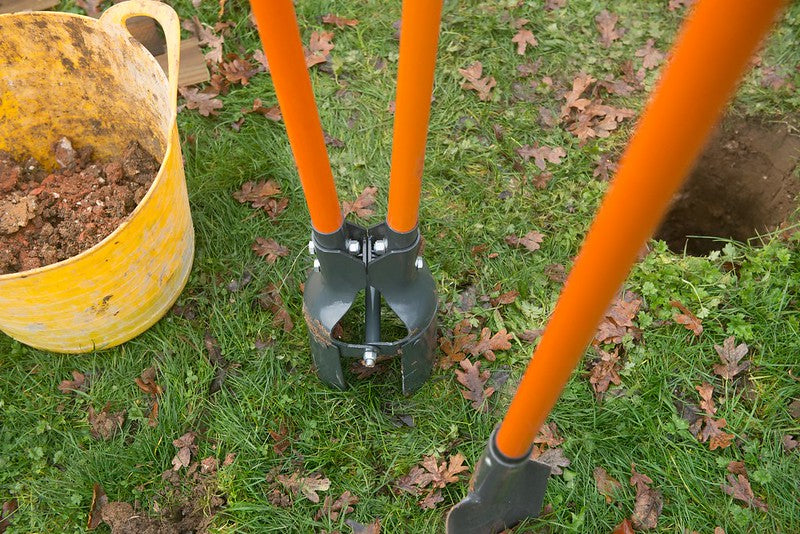The photograph captures an outdoor scene, likely in an open yard or field, showcasing various gardening equipment. The ground, covered in green grass and scattered with dry brown autumn leaves, displays the results of some active work. Positioned centrally are a pair of yellow-handled posthole diggers, resembling two shovels joined in a scissor-like fashion, designed for digging neat, cylindrical holes. To the upper right of the image is one such neatly dug hole, surrounded by dark brown earth, indicative of recent disturbance. The exact depth of the hole is ambiguous due to shadow play. To the left, a yellow bucket filled with red and brown dirt sits beside the tools. An additional digging implement with an orange handle and a narrow, possibly spade-like, silver head lies in the immediate foreground, suggesting it might be used for further refinement of the holes. The overall scene suggests an ongoing task of preparing the ground, likely for planting or construction.